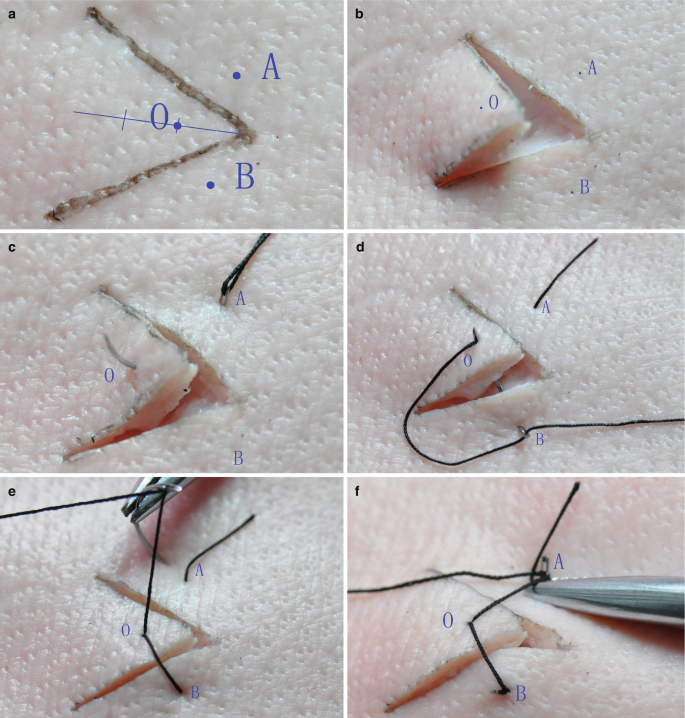The image illustrates a step-by-step guide on how to stitch a V-shaped cut, potentially on human skin or a skin-like material, across six different labeled boxes: A, B, C, D, E, and F. These close-ups detail the intricate process, starting with the largest, more visible triangular cut in box F. Box F features tweezers holding the skin and the beginning of the threading process. Box E showcases an intermediate step where the thread is partially in place. In box D, the thread is shown crossing over the wound, stitching it closed. Box C highlights further progression of the stitch, displaying the threading technique more clearly. Box B, however, interestingly does not show any thread, adding a layer of complexity to the instructional sequence. Lastly, box A includes markings next to the V cut labeled "A" and "B" to guide where the needle should enter and exit, illustrating the final, closed wound with black thread. The beige-pink tone of the material used suggests a simulation of white human skin, possibly for medical training purposes.